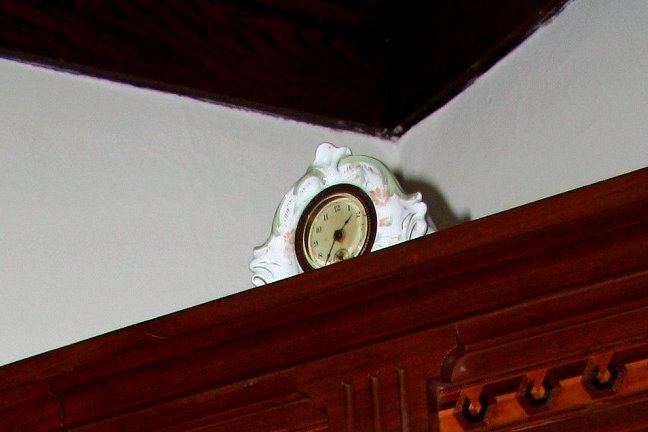This photograph depicts the top of a large, antique wooden cabinet stretching across a corner of a room. The cabinet's reddish-orange wood paneling complements its vintage charm. The viewpoint is angled upwards towards the point where two white walls converge at the ceiling, which features a dark mahogany trim.

Sitting atop the cabinet is a distinctive, ornamental clock encased in a curved, ornate white housing with wave patterns reminiscent of ceramic or china. The outer housing is adorned with hints of green and white, accentuated by touches of pink flowers on either side. The clock itself, with its beige face, is encircled by a faded brown rim.

The analog clock, which shows the time at approximately 1:35, displays black numerals and hands. The lack of background elements and the clock’s shadow cast against the stark white backdrop emphasize its prominence in the image.